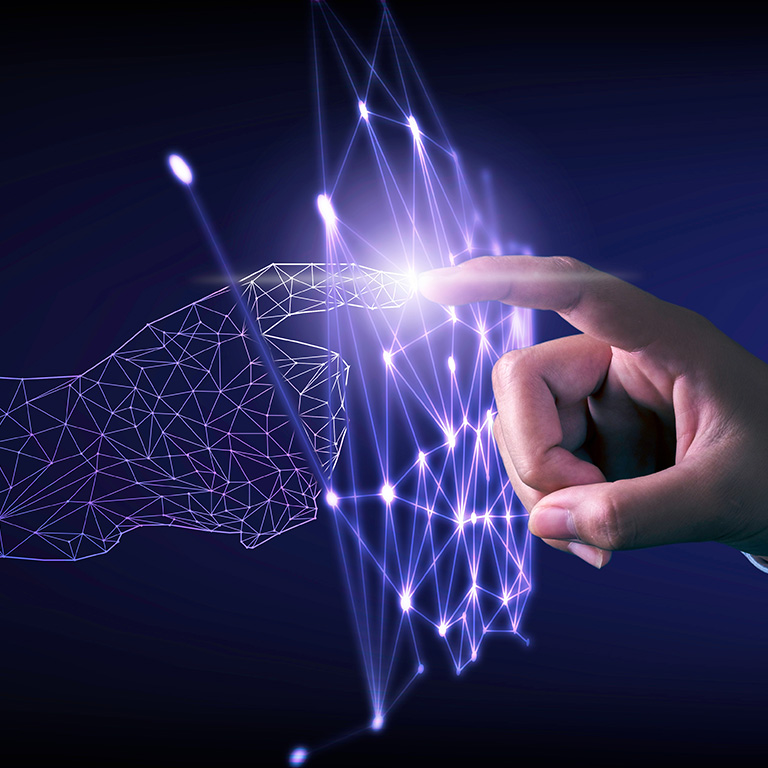In this computer-generated digital artwork, set against a purplish-black background, we see a striking juxtaposition between a realistic human hand on the right and a 3D modeled hand composed of neon purple vertice lines on the left. These lines form the shape and suggest the movement capabilities of the digital hand. The two hands are reaching towards each other, their extended fingers almost touching in a focal point of luminous white light. The connecting area between the fingers is further detailed by a web of interconnected vertice lines and illuminated dots, creating a vivid point of connection and merging. This glowing intersection is highly reminiscent of Michelangelo's famous "The Creation of Adam," emphasizing the symbolic bridge between the human, the digital, and the artificial within a matrix-like environment.